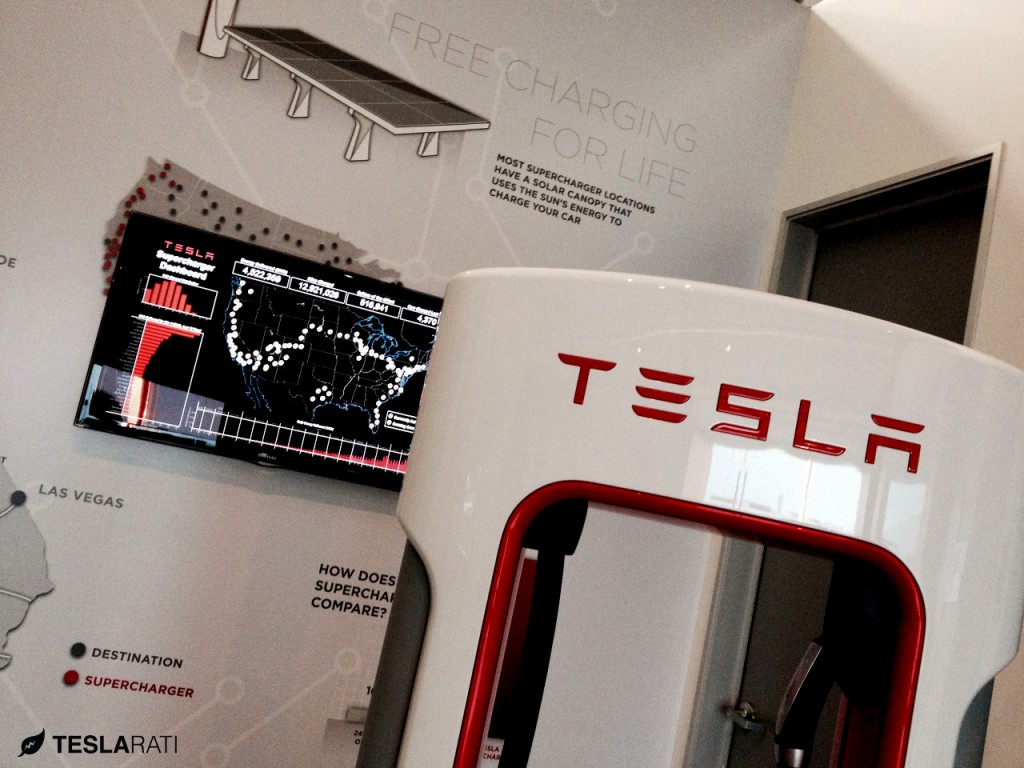The image depicts a Tesla charging station prominently in the foreground, adorned with the iconic Tesla logo in red on a sleek white structure. The charging station is situated next to a white wall with bold red lettering that reads "Free Charging for Life." The wall also features a map of the United States illuminated with pinpoints, likely indicating Tesla Supercharger locations across the country. On the left side of the image, there appears to be a solar panel, emphasizing the use of solar canopies in most Supercharger locations to harness the sun's energy for vehicle charging. The background includes an open door, seemingly leading from a garage into a house, enhancing the domestic context of the scene. Also visible on the wall is a TV displaying the Tesla Supercharger Dashboard with numbers and pinpoints, further detailing the Supercharger network. The overlay text "Tesla Roddy" alongside a leaf adds an editorial element to the photograph. The overall atmosphere suggests a blend of cutting-edge technology with everyday usability, centered around Tesla's innovative charging infrastructure.